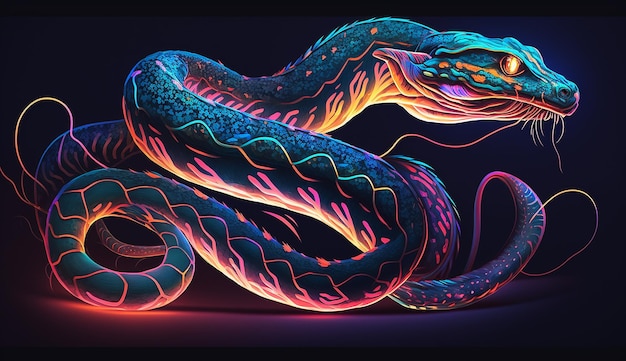This captivating illustration features a deadly-looking, stylized snake set against a black background that transitions to purple at the bottom. The landscape-oriented image, approximately five inches wide and three inches high, showcases the snake with a glowing, electrified appearance. The snake's head, situated in the upper right corner and facing right, has a large, golden pupil with white whiskers extending from its mouth. The top of the head is adorned with green and blue lines and orangish dots beneath the eye, leading to pink lips at the nose tip.

The snake's body, primarily electric blue with sections transitioning into dark purple, is decorated with bright neon magenta, orange, and yellow markings. These fiery colors streak along its length, creating a vivid, fluorescent effect. The underbelly, starting orange and shifting to pink, features branch-like patterns with outcroppings of magenta.

A thin ridge of light green spikes runs down the snake’s back, contrasting with glowing gold and orange effects underneath and along the body. The snake's extensive, coiled form loops throughout the image, eventually tapering into a thin magenta wisp just below its head. This intricately detailed, color fantasy illustration masterfully depicts the snake's vibrant, luminous essence.